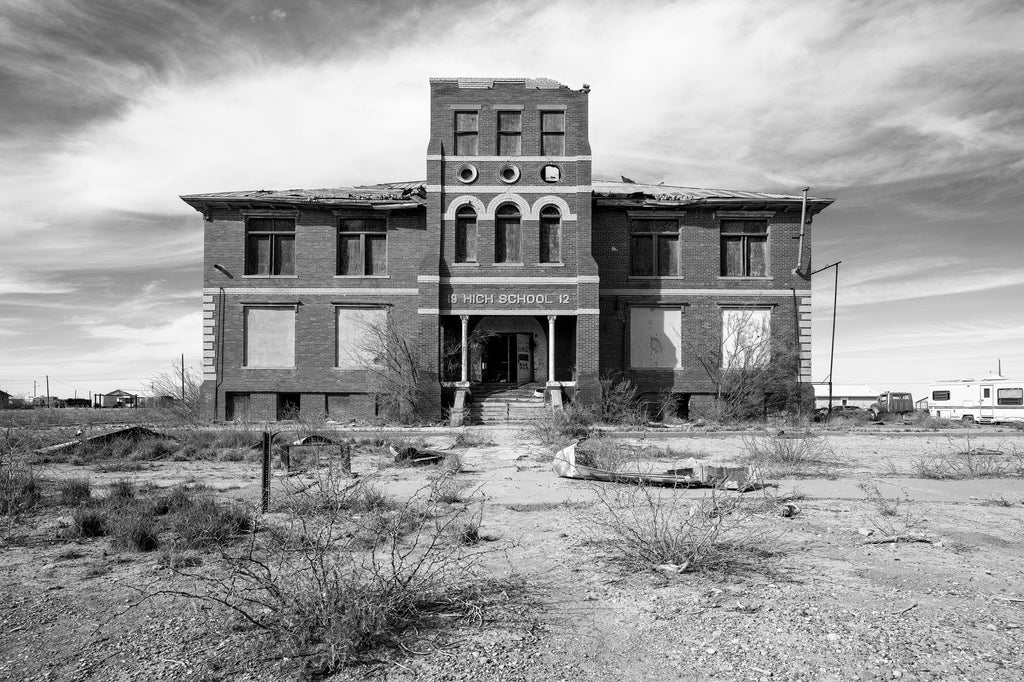The black and white photo captures a hauntingly desolate, two-story brick high school, abandoned and out in the middle of what appears to be a desert. The facade, which reads “19 High School 12,” suggests it was built in 1912. A partially collapsed, rotting roof and boarded-up windows dominate the scene, with wooden boards covering many of the windows across both floors and possibly the basement. Prominent architectural features include three arches above the main entrance and some pillars, although the front door seems to have been forced open at some point, hinting at signs of trespass over the years.

The exterior grounds are barren, strewn with debris, dirt, sand, and weeds, creating a stark contrast against the once-thriving educational institution. To the right of the building, there is a camper and a truck cab parked nearby, indicating perhaps temporary refuge or abandonment. The left side of the background shows distant, indistinguishable buildings. Despite the dilapidation, the structure suggests it was once a notable and sturdy establishment, now reduced to a relic of a bygone era.